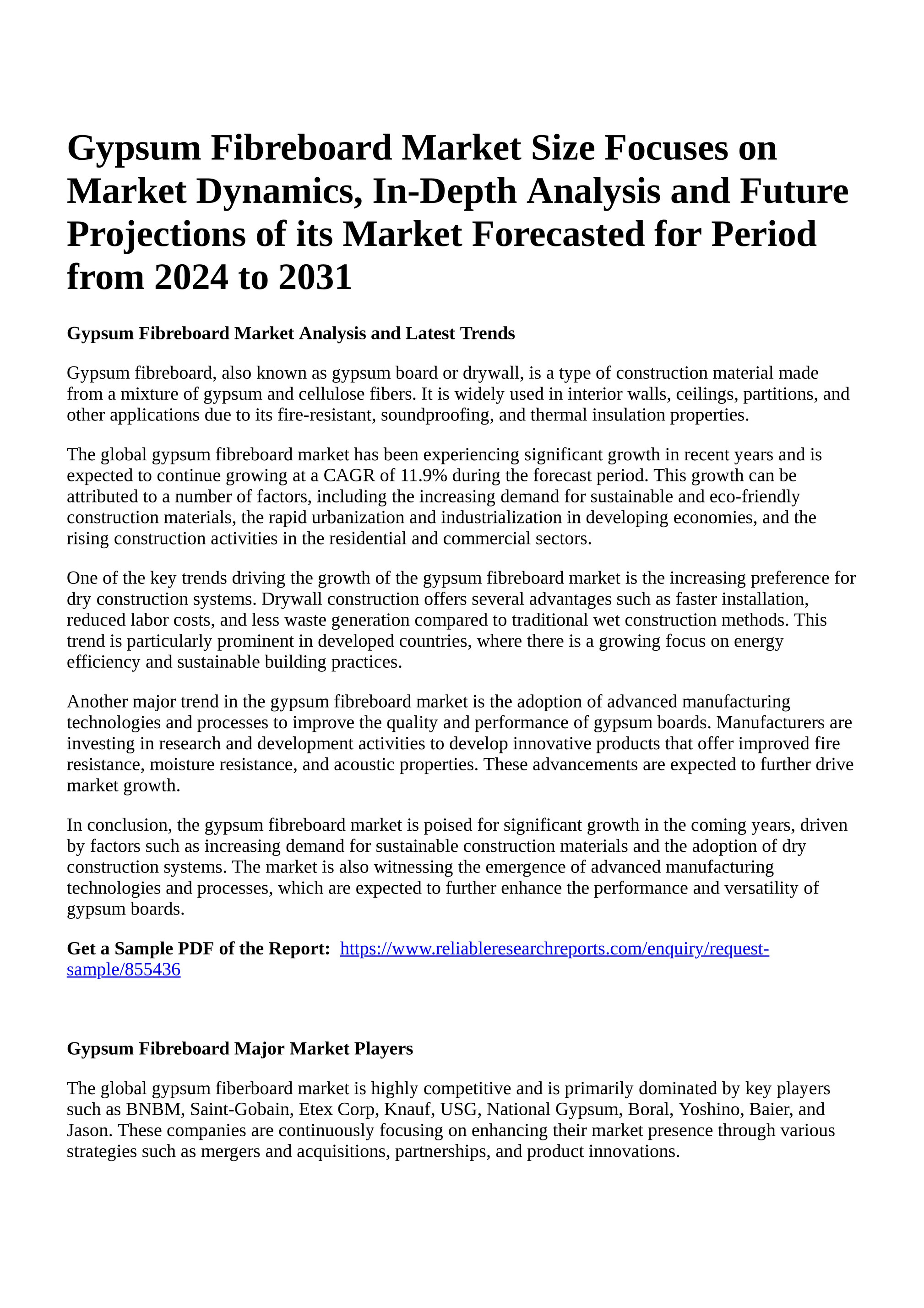The image depicts an online market forecast article titled “GYPSUM FIBER BOARD MARKET SIZE: Focusing on Market Dynamics, In-Depth Analysis, and Future Projections from 2024 to 2031.” The article begins with a detailed explanation beneath a bolded subheading, "GYPSUM FIBER BOARD MARKET ANALYSIS AND LATEST TRENDS." It describes Gypsum Fiber Board, also known as Gypsum Board or Drywall, as a construction material made from a mixture of gypsum and cellulose fibers. This material is praised for its widespread use in interior walls, ceilings, partitions, and other applications due to its fire resistance, soundproofing, and thermal insulation properties. The article mentions the significant recent growth of the global gypsum fiber market, projecting continued expansion at a CAGR of 11.9% due to rising demand for sustainable and eco-friendly construction materials. Visually, the article's layout features black text on a white background, with accents of blue towards the bottom where a clickable hyperlink invites readers to obtain a sample PDF of the report. The content of the article spans from top to bottom, thoroughly detailing the various aspects of the gypsum fiber board market.